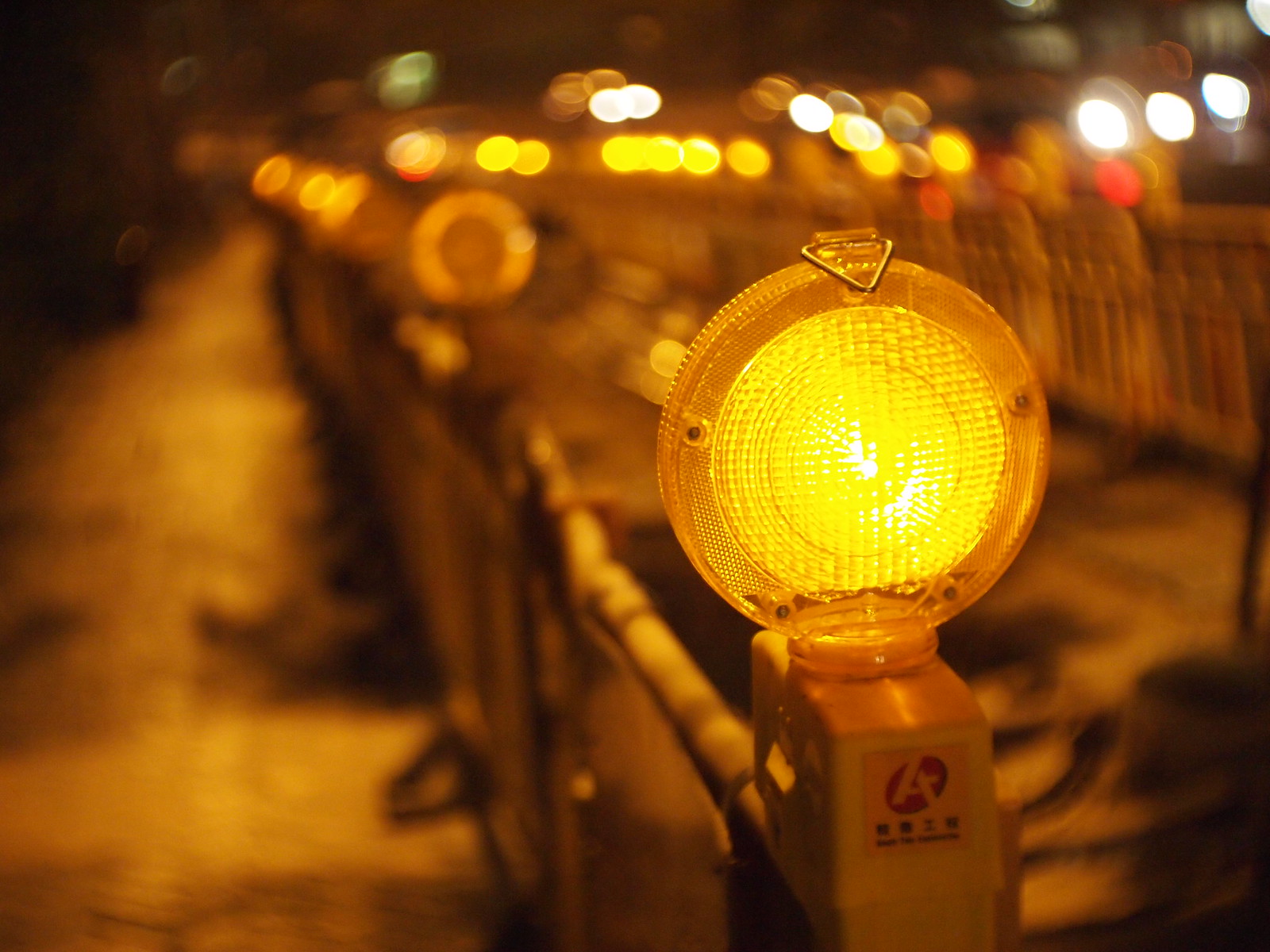The outdoor photograph captures a nighttime scene with a distinct amber hue permeating the surroundings. It focuses on a close-up view of a round, amber-colored safety light mounted on a post, which is textured with small squares and firmly attached to a series of temporary highway barriers. These barriers, likely silver and metallic, might be surrounding a potentially hazardous hole in the ground, indicated to prevent pedestrians from nearing it. The illuminated safety light in the foreground is sharply in focus, casting a yellow glow that highlights the attached bars and fence sections. As the eye moves further back, additional identical lights can be seen, although they appear increasingly blurry and less brightly lit. Scattered among the yellow lights are some gold, green, and white circles, with two distinct red safety lights also visible on the barriers. On the right side of the image, a second set of barriers can be distinguished. The background fades into complete darkness, with only the barriers and the lights visible, adding to the atmosphere of a dimly lit, possibly construction-related scene. Adjacent to the barricades, a sidewalk made of tile or cobblestone can be noted, further establishing the setting as a precautionary zone amidst a nighttime streetscape.